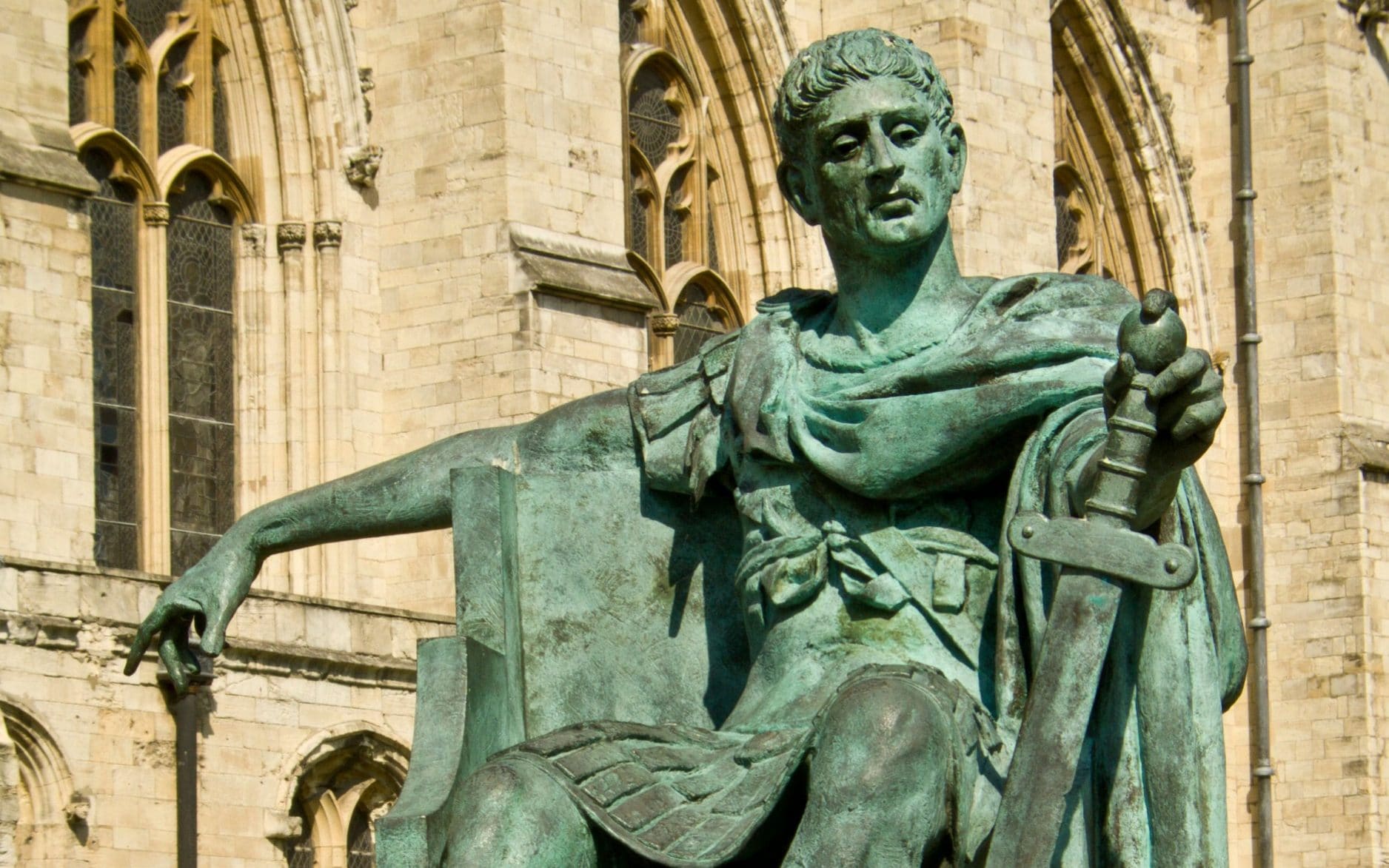The image features a green-hued statue, likely made of a copper compound that has undergone oxidation. The statue, reminiscent of a European sculpture from around the 15th century, depicts a warrior or commander seated on a throne-like chair. The figure is donning period-appropriate attire, complete with a cape and traditional warrior dress. He has a large sword in his left hand and appears to be contemplatively gazing down at it, his expression one of indifference or thoughtfulness. Behind the statue stands a large brick building, possibly a medieval church or government structure, characterized by its natural stone walls, stained glass windows, and distinctive arches above the windows. The scene is illuminated by daylight, casting shadows that emphasize the statue's aged and weathered features.